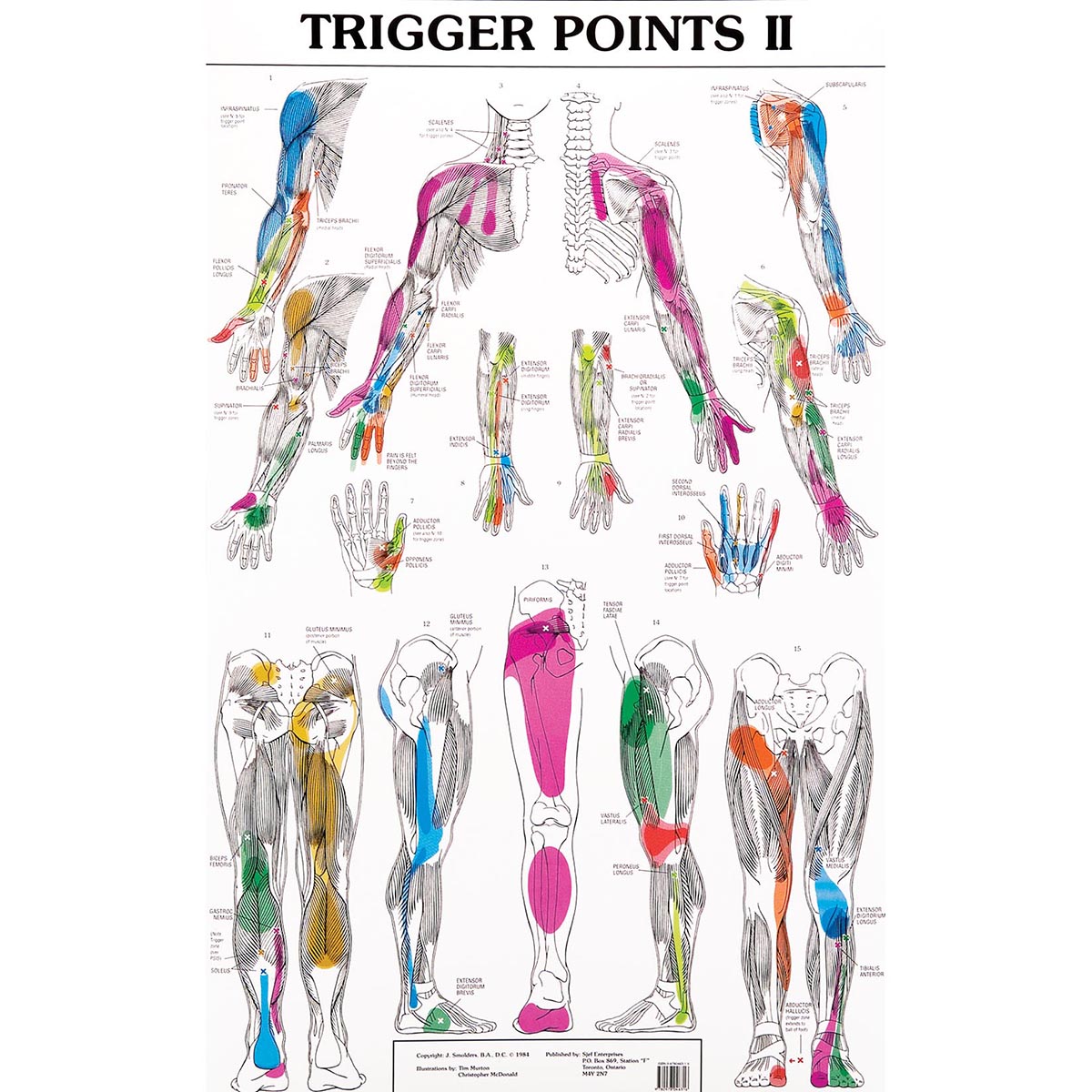This diagram, labeled "TRIGGER POINTS II" in bold black font at the top, serves as an informative poster on musculoskeletal anatomy focusing on trigger points. It is visually structured to represent a human body, starting with the chest, arms, and hands at the top, progressing to the legs, knees, and feet at the bottom. Each body part illustrated—from the back of a leg to the various angles of arms and hands—is marked with specific areas highlighted in a variety of colors including pink, blue, green, orange, red, and yellow. These colors presumably denote different trigger points or levels of pressure. Despite the small and pixelated labels that render specific text unreadable, the diagram is rich in detail. At the bottom, there is a rectangle containing copyright information, a barcode, and references to publication, suggesting the image may originate from a textbook or scientific resource.